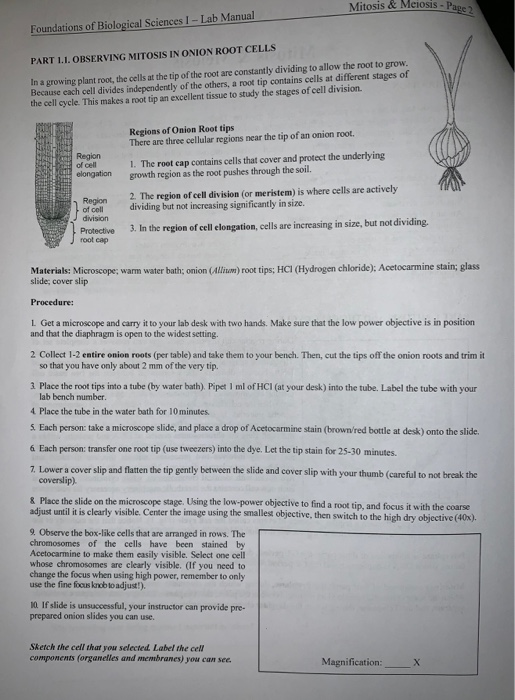This image depicts page 2 of the "Foundations of Biological Sciences 1: Mitosis and Meiosis" lab manual. The page is titled "Observing Mitosis in Onion Root Cells," and outlines the aim and procedure of a laboratory experiment designed to study cell division. The text emphasizes that the cells at the tip of a growing onion root are in a constant state of division, making this an ideal tissue for observing different stages of the cell cycle. The page is written in black and white and includes detailed sections on the three cellular regions near the root tip: the protective root cap, the region of cell division, and the region of cell elongation. The necessary materials listed include a microscope, water bath, onion root tips, and HCI, among others. The page is quite detailed, including step-by-step procedural instructions for conducting the experiment.